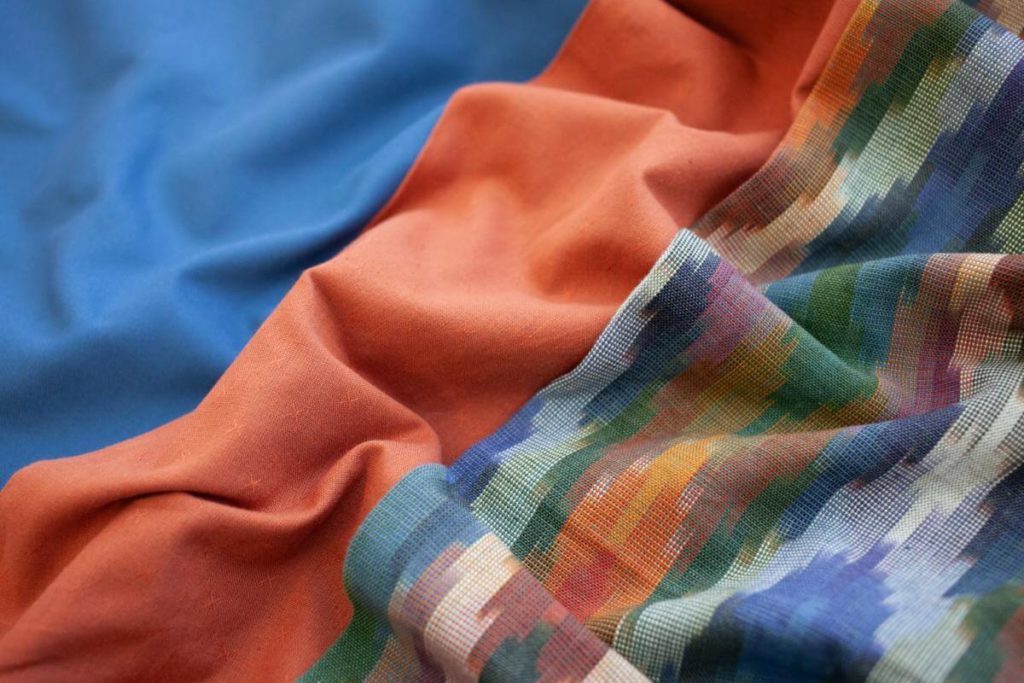The image features a close-up view of three distinct pieces of fabric, arranged in a diagonal layout. The upper left section showcases a solid blue fabric with visible wrinkles, suggesting it could be a sheet. A narrow, folded strip of vibrant coral fabric runs diagonally from the upper right to the lower left, adding a splash of color to the composition. In the lower right corner, a larger piece of fabric with a rougher texture displays a complex, multicolored pattern. This fabric includes an array of hues such as orange, brown, green, light green, blue, light blue, and possibly coral, woven together in tiny square patterns. The fabrics appear to be overlapping, creating a layered, informal arrangement that emphasizes their varied textures and colors. There are no borders or text in the image, keeping the focus entirely on the detailed, colorful fabrics.